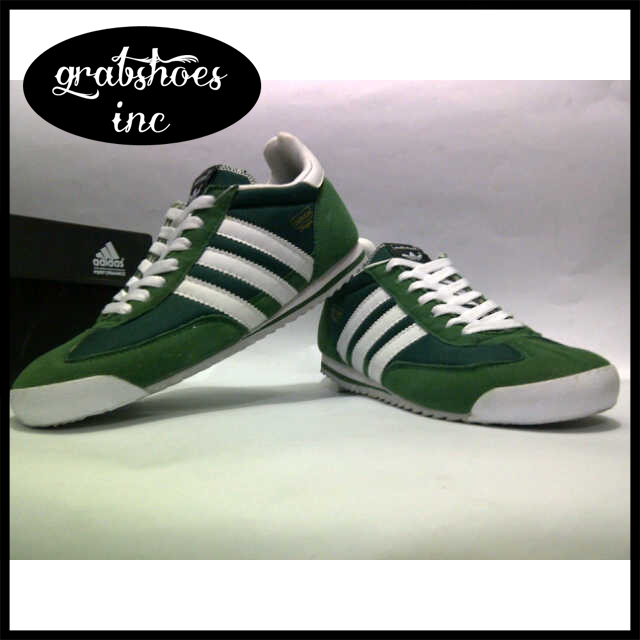The photograph, which appears to be an advertisement, features a centrally-placed pair of new, green Adidas running sneakers with distinctive white stripes, laces, and soles. One shoe has its heel propped on the foothold of the other. The shoes are positioned on a curved white paper surface, against a white background that subtly transitions into an off-white or light gray. In the upper left corner of the image, there is a black oval with the text "Grab Shoes, Inc." written in white, cursive-like lowercase letters. A portion of a black shoebox with the white Adidas logo is visible in the back left of the composition. The entire photograph is framed by a black border.